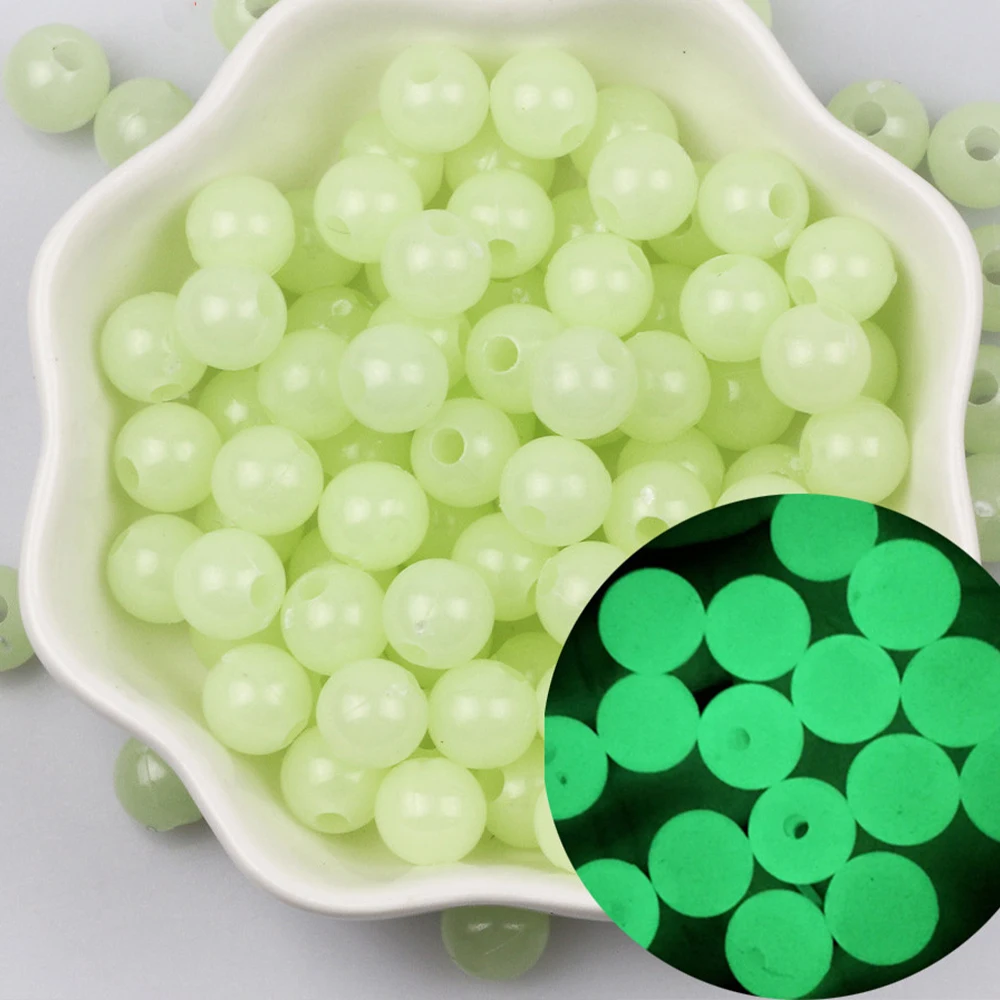This photograph captures a detailed top-down view of a uniquely shaped, white ceramic bowl resembling a flower, sitting on a white table. The bowl is filled with iridescent, shiny beads that spill over onto the table around it. Each bead has a hole in it and appears white with a light green tint, suggesting they might glow in the dark. In the lower right corner of the image, there is a superimposed visual showing these same beads glowing bright green against a black background, indicating their luminous properties. This striking composition contrasts the bowl's refined porcelain texture with the beads' vibrant, almost wet appearance, providing both a daytime and nighttime perspective of these intriguing, potentially Halloween-themed decorations.